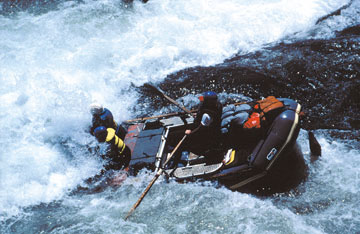In this thrilling image of a whitewater rafting adventure, a black raft is shown battling through violent, frothy rapids. The raft, which is tilted and nearly submerged at the front, holds three people all clad in life jackets and helmets—two in the front, and one person commanding the oars at the back. The river water, splashing vigorously, is so forceful that it completely engulfs the front segment of the raft. A prominent rock juts out in the middle of the screen, with the raft navigating along its bottom edge into the rushing currents from the top. A metal frame bar, attached to a large tote, is visible in the middle of the raft, and several life jackets are secured at the rear. The action is set against a backdrop of aggressive waters and a rock bank, indicating this is likely a high-level, challenging stretch of river, possibly a Class V rapid. The intense motion captured and the detailed gear of the rafters underscore the demanding and exhilarating nature of this daring outdoor escapade.